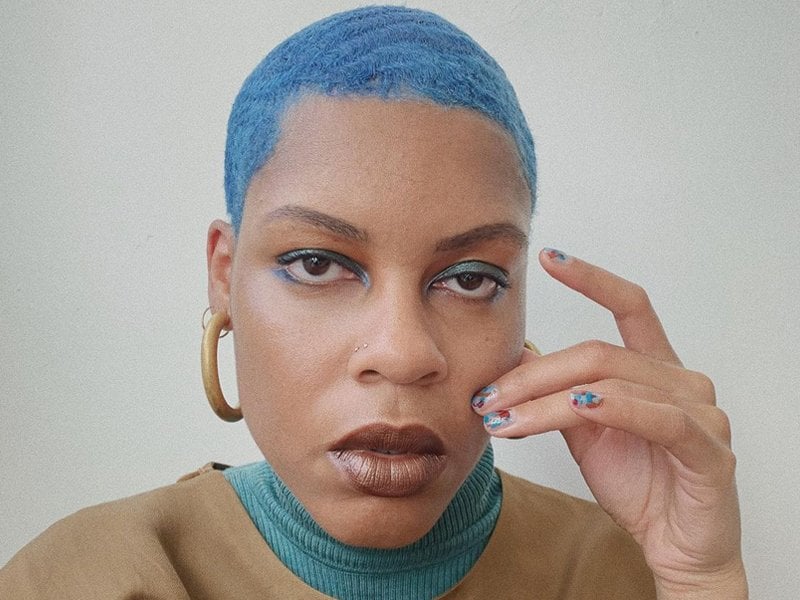The image features a close-up of an African-American woman, staring directly at the camera with an expressive and intense gaze. She has striking, vibrant blue short hair that complements blue eyeliner accentuating her brown eyes, which are framed by brown eyelashes and eyebrows. Her lips are full and adorned with a subtle brownish-red hue with a slight golden shine. 

She is pinching her left cheek with her hand, displaying fingernails that are intricately painted in a mix of blue, red, and white nail polish. The woman wears large, hooped earrings that appear to be golden, adding a bold accessory to her appearance. Her attire consists of a beige shirt layered over a turquoise blue turtleneck, lending a fashionable contrast to her outfit. 

She also has two small circular piercings on her right nostril, adding to the details of her facial adornments. The background is a simple, flat gray which highlights her striking appearance, keeping the viewer’s focus on her. The composition of the image only shows her from the shoulders upward, ensuring that her face and accessories are the focal points.